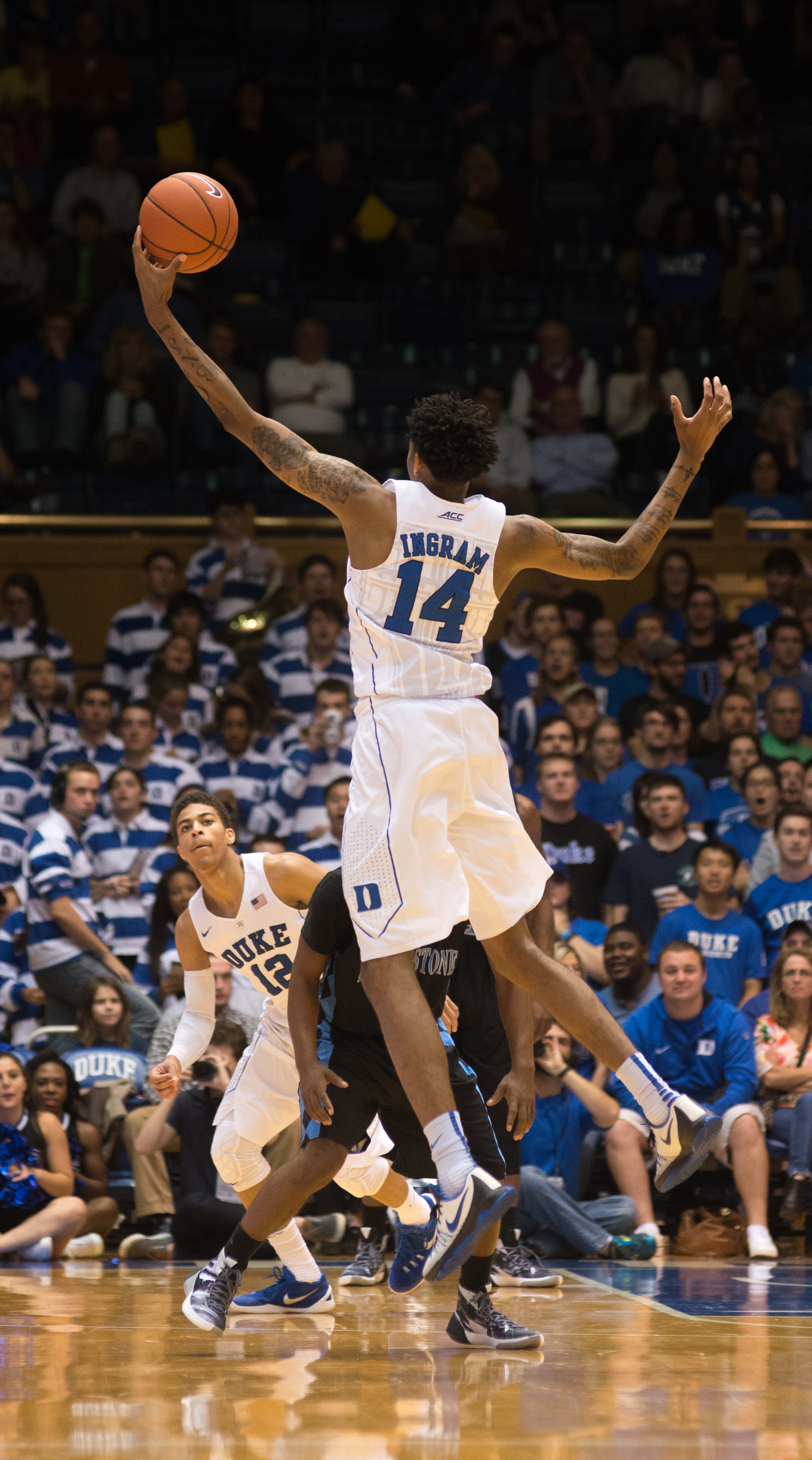The photograph captures a high-intensity moment during an indoor basketball game in a stadium. The focal point is Ingram, an African American player wearing a white uniform with blue lettering that reads "Ingram 14" on the back. He is mid-air, leaping to grab the basketball with his left hand. His uniform, which includes blue and white socks and shoes, also carries the ACC logo. Ingram’s black tattoos are visible on both arms. Directly in front of him is a player in a black and blue uniform with "Stone" partially visible on the back. This opposing player is facing the camera, while Ingram faces away. To the right of Ingram, another Duke player, number 12, wearing the same white and blue uniform, is grounded on the polished hardwood court. The background is filled with spectators; those in the front rows are dressed in Duke’s team colors, with some wearing striped blue and white tops, while higher up, fans are dressed in regular attire, reflecting a vibrant and supportive atmosphere.